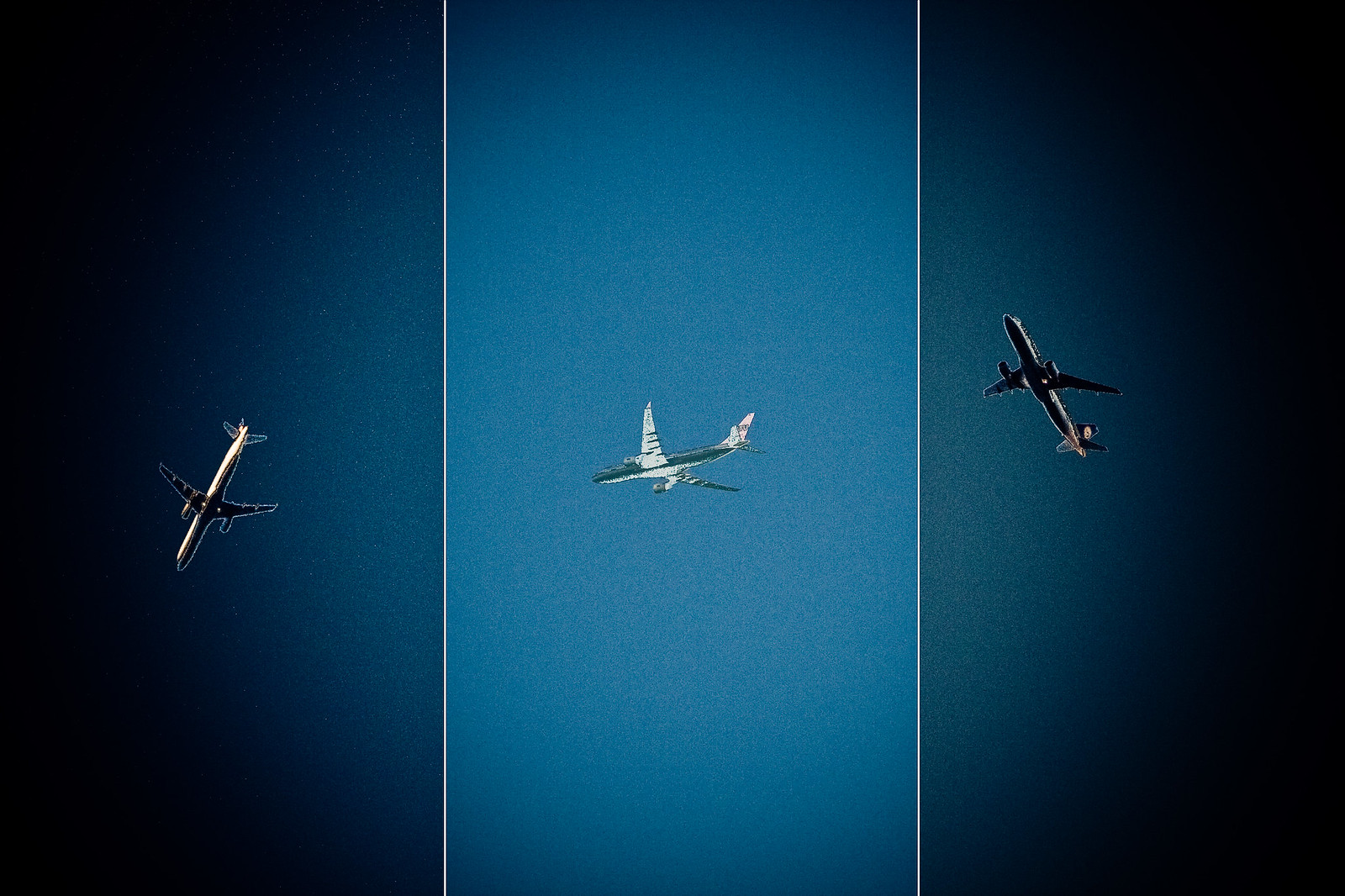This art piece is a captivating compilation of three tall, narrow rectangular photographs of airplanes in flight, arranged side by side to form a single cohesive circle, evoking the view through an eyepiece of a camera or telescope. Each panel features a gradient blue sky, with the left and right panels transitioning from dark to lighter blue towards the center, enhancing the circular effect.

The left panel showcases a large commercial airliner, captured from below, angling downwards with its nose pointing to the bottom left, adding a dramatic sense of descent. The center panel, featuring a smaller personal aircraft, presents a lighter blue sky backdrop and depicts the plane in a slightly downward-tilted side profile, flying towards the left. Lastly, the right panel presents another large commercial jet ascending upwards with its nose directed towards the top, captured from a low angle that reveals the plane’s belly.

The borders of each photograph are shaded in black at the corners—top left, top right, bottom left, and bottom right—giving the impression of shadows, further focusing attention on the dynamic compositions of the aircraft within the circular frame. Together, the three images create a visually striking piece that draws the viewer into a varied yet harmonious portrayal of aviation from multiple perspectives.